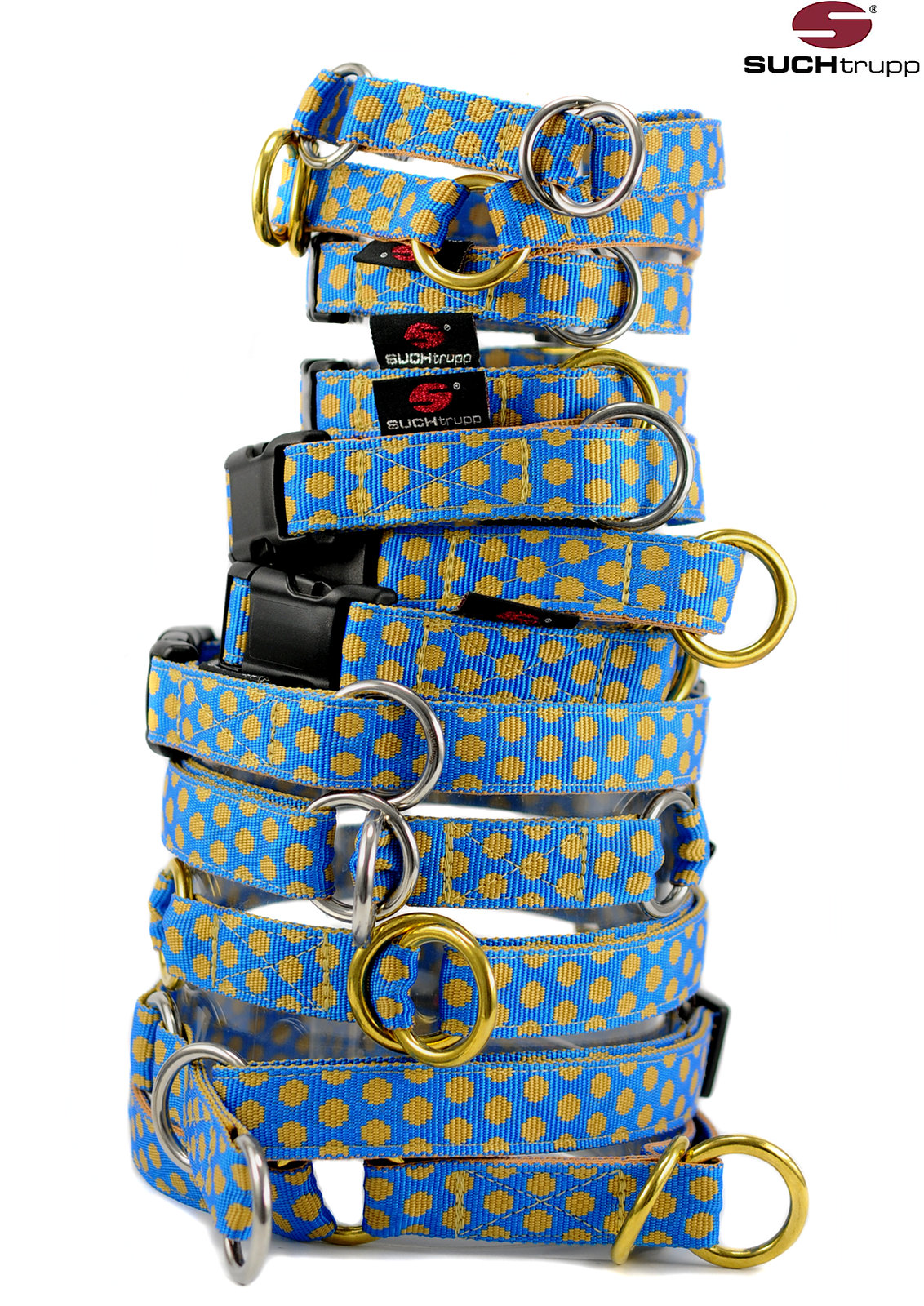In the photo, against a white background, there is a logo in the upper right corner featuring the maroon letter "S" with a small trademark symbol beside it, and the brand name "Suchtrup" written in black letters. Below the logo, there is a neatly stacked assortment of twelve dog collars incrementally decreasing in size from bottom to top. Each collar is primarily blue with distinctive golden or yellow polka dots and features a black fabric tag bearing the same "S" logo as in the upper right corner. The collars are designed with either gold or stainless steel clasps. All the collars use a clicking latch mechanism and are adorned with rings for leash attachment.